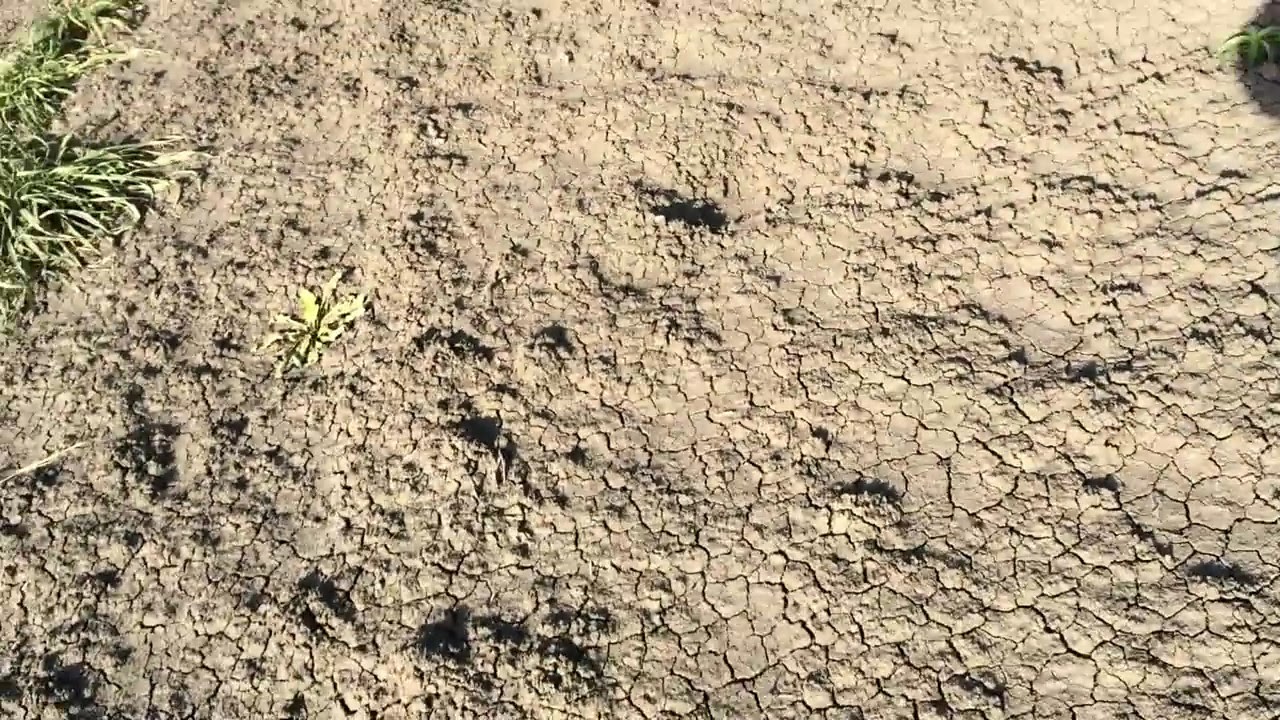This detailed outdoor photograph showcases a close-up view of a dry, arid ground bed occupying the entire frame. The earth is light brownish-tan, deeply cracked, and reminiscent of parched dirt or clay, forming an intricate, almost checkerboard-like pattern of rectangular and square shapes. Prominently in the center of the image, lightly indented paw prints, possibly from a cougar or wolf, add a hint of life to this otherwise barren landscape. The ground is nearly bare, with sporadic black patches indicating extreme dryness and lack of moisture. In the upper left corner, a small cluster of desert vegetation struggles to thrive, with a tiny bit of green grass visible, echoing the dryness and hostility of the environment. The upper right corner also hints at a small fragment of grass, but overall, the photograph captures the essence of a harsh, dessicated terrain devoid of human or animal presence.